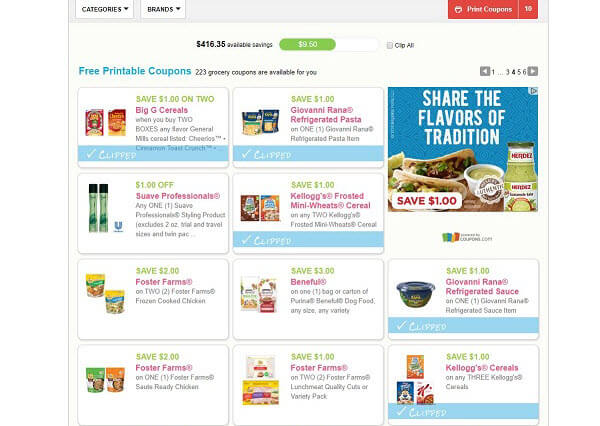This image depicts a square-shaped page filled with various food items and an assortment of free printable coupons. The detailed breakdown of the available coupons is as follows:

1. Save $1.00 on two Big G cereals when you buy any two boxes, any flavor, from the General Mills cereal range.
2. Save $1.00 on Giovanni Rana refrigerated pasta.
3. Save $1.00 on any one Suave Professionals styling product (excludes 2-ounce, trial, and travel sizes).
4. Save $1.00 on Kellogg's Frosted Mini-Wheats Cereal when you purchase any two boxes.
5. Save $2.00 on Foster Farms when you buy any two Foster Farms Frozen Cooked Chicken products.
6. Save $3.00 on Beneful pet food.
7. Save $1.00 on Giovanni Rana refrigerated sauce.
8. Save $1.00 on any Kellogg's cereals.
9. Save $1.00 on Foster Farms products.
10. Save $2.00 on certain Foster Farms items.
11. An advertisement for the Eres brand featuring the tagline "Share the flavors of tradition" and offering a $1.00 savings.

The image combines vibrant visuals of food products with the practicality of money-saving opportunities through easily accessible coupons.